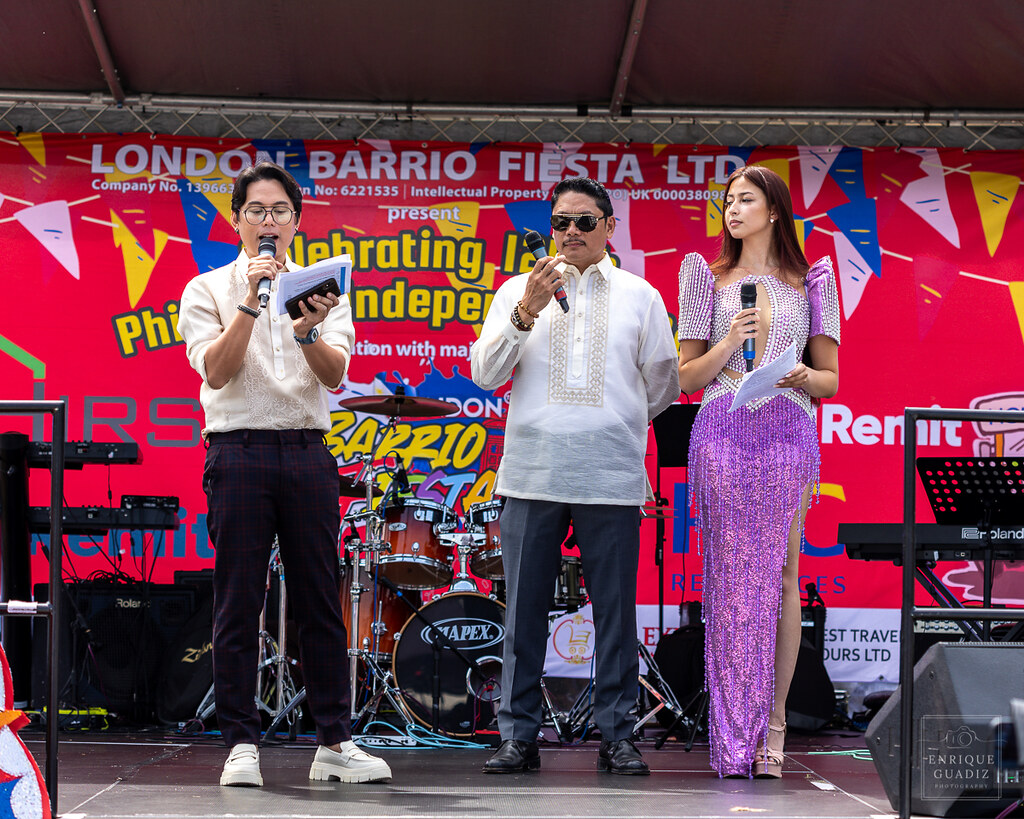The image captures an outdoor festival scene in full color during the daytime, featuring three individuals standing on a stage. Positioned on the left is an Asian man with dark hair and round glasses, dressed in a white shirt, black pants, and white shoes. He holds a microphone in one hand and a piece of paper in the other, appearing to speak into the microphone. The central figure is also a man, possibly Asian, identified by his dark hair and darker features. He is wearing sunglasses, a cream-colored shirt with a subtle design, gray dress pants, and black shoes. The woman on the far right, identified as Asian, has dark brown hair and is dressed in a striking purple and white sequined dress, paired with high-heeled sandal shoes. She too holds a microphone. The backdrop features a large, vibrant red banner adorned with additional colors like yellow, blue, white, and pink. Although partially obscured by the individuals, the visible text on the banner reads, "London Barrio Fiesta Limited presents," followed by additional text that remains unreadable due to their positioning. There is a set of drums visible behind the three people, enhancing the festive atmosphere of the scene.